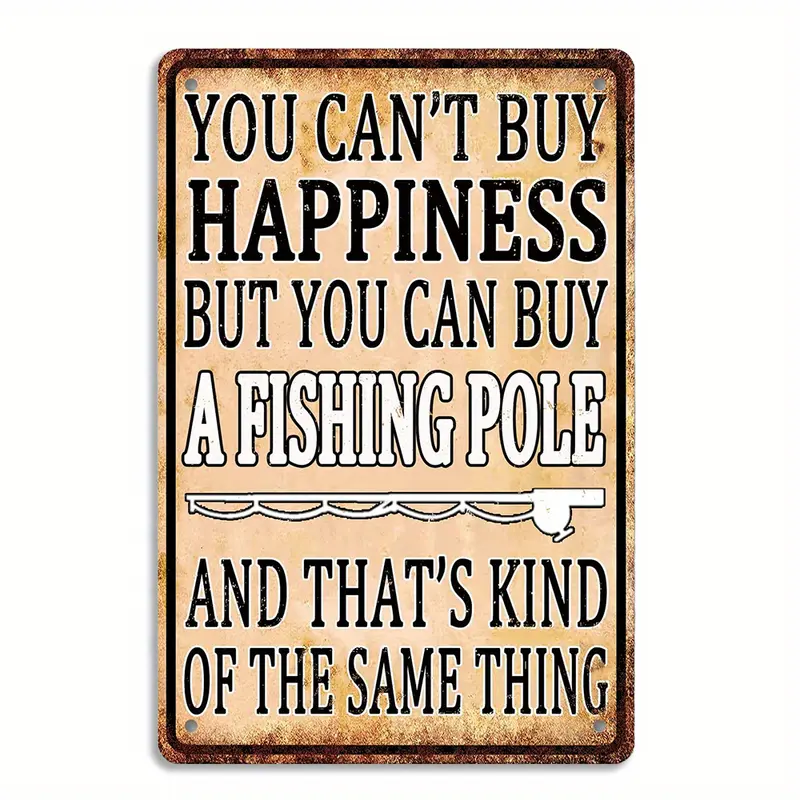The image is of a rustic, beige, rectangular sign bordered by a thin, black, rounded-edge contour. The sign exhibits patches of rust, particularly at the top and bottom edges, adding an aged appearance. At the top, black text encased in a white outline reads, "You can't buy happiness but you can buy." Directly beneath this, the phrase "a fishing pole" is prominently displayed in white text. Just below the text, there is a white silhouette outline of a fishing pole, angled to the left. The pole is detailed with elements including a reel on the right side and lines curving downwards to suggest threads and waves. At the bottom of the sign, black text humorously concludes, "and that's kind of the same thing." The sign has small gray holes in all four corners, presumably used for mounting. The combination of beige color, black contour, white and black text, and rust details give the sign a vintage, weathered look.